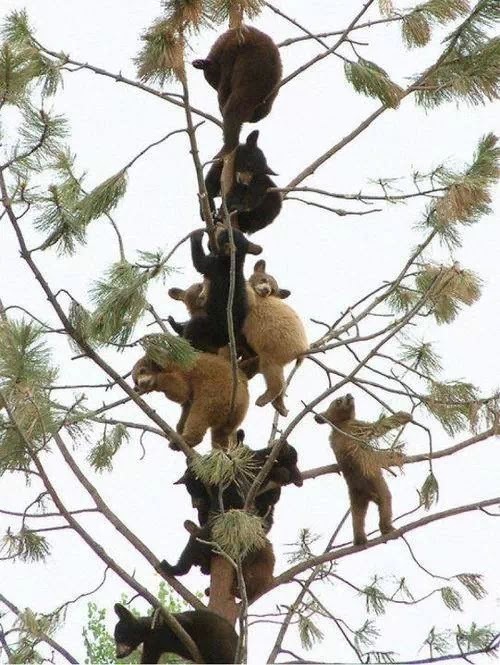This photograph depicts a tall, slender pine tree with thin branches sparsely adorned with pine needles, set against a stark white sky. The tree is intriguingly covered with approximately 10 to 12 bear cubs of various colors, ranging from light tan to dark black. These endearing little creatures are scattered along the trunk and branches, creating an almost vertical line as they cling, rest, and nestle amongst each other. The sight of these cubs, many of whom seem to be cuddling or sleeping on the branches, is both fascinating and surreal, almost reminiscent of a CGI or AI-generated image. One curious bear cub is exploring near the bottom right of the tree, slightly apart from the others who form a dense cluster that accentuates the tree's height and slenderness.